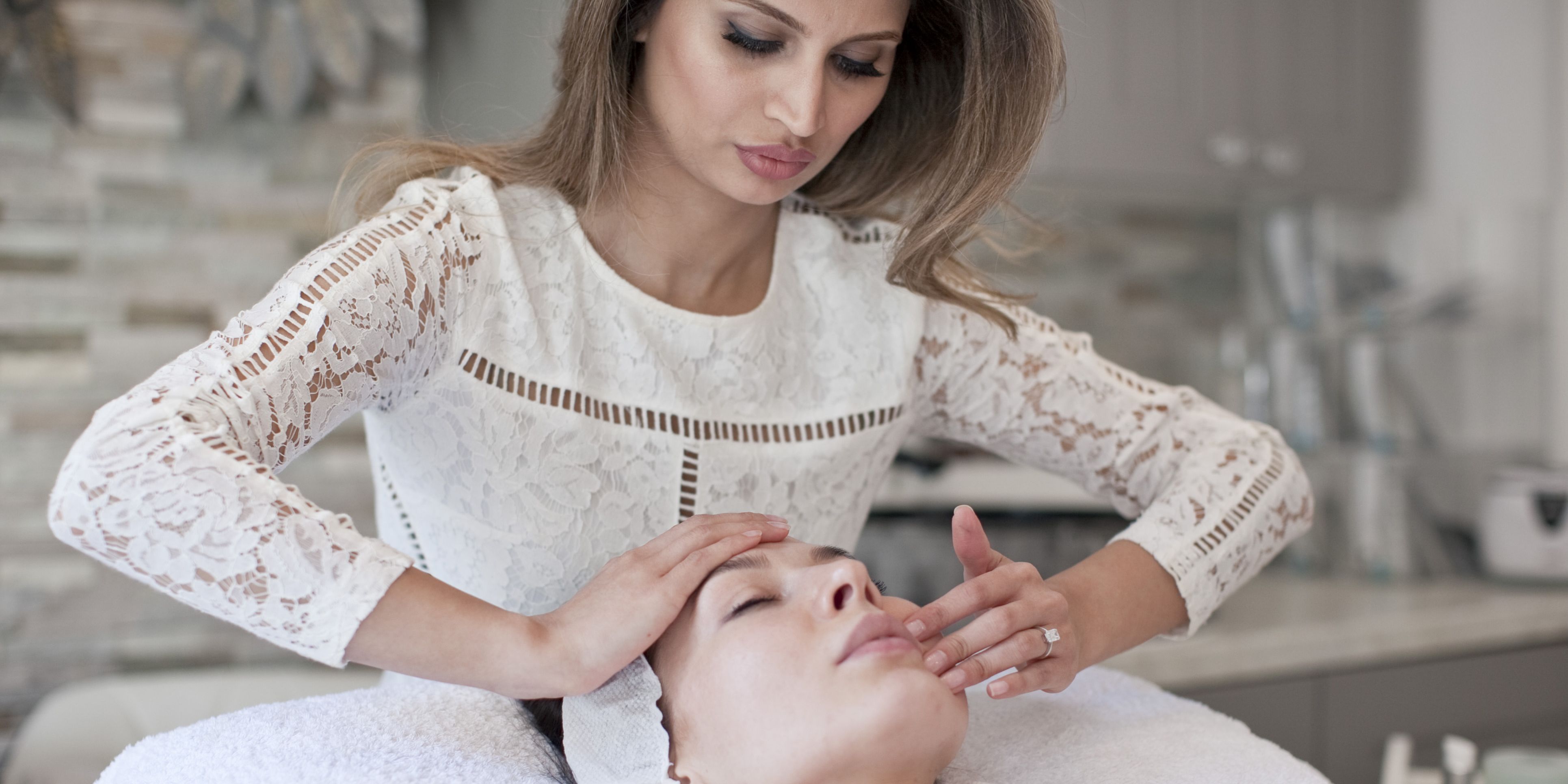In this photograph, a serene scene unfolds where a woman is receiving a soothing facial massage. She is lying down with her head cushioned by a white pillow or towel, eyes closed in a state of tranquility. Only her head is visible, framed by a soft, white surface. The woman administering the massage has long brown hair and wears an elegant, lacy long-sleeved blouse or dress. She is deeply focused, with one hand gently resting on the client's forehead and the other tenderly touching her lips and chin area. This therapist, possibly Middle Eastern in descent, wears strong makeup, a wedding ring, and exudes professionalism and care. The background is softly blurred, revealing indistinct hints of a marble countertop and gray cabinets, adding to the peaceful ambiance of the spa-like setting.